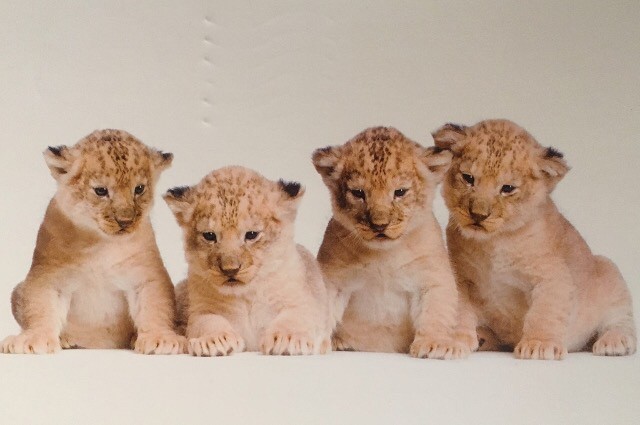The photograph captures four lion cubs positioned next to each other on a simple white surface, all appearing to be around eight to ten weeks old. The photo seems to be an image of an existing print, which shows slight damage with indentations on the top middle section. The cubs, soft and fuzzy, with fur that is primarily a soft tan blending into a golden hue, have distinct markings on their heads. These markings, resembling lines that form spots, create a pattern of light brown and dark brown spots on their rounded heads. The lion cubs' ears feature tiny tufts and conspicuous black or dark brown fuzz on the back. Their endearing, large paws are prominent, showing hints of small claws. While three of the cubs look inward, the leftmost one gazes down and to the right. Their charming large heads and relatively small eyes give them a particularly adorable appearance against the stark white background.